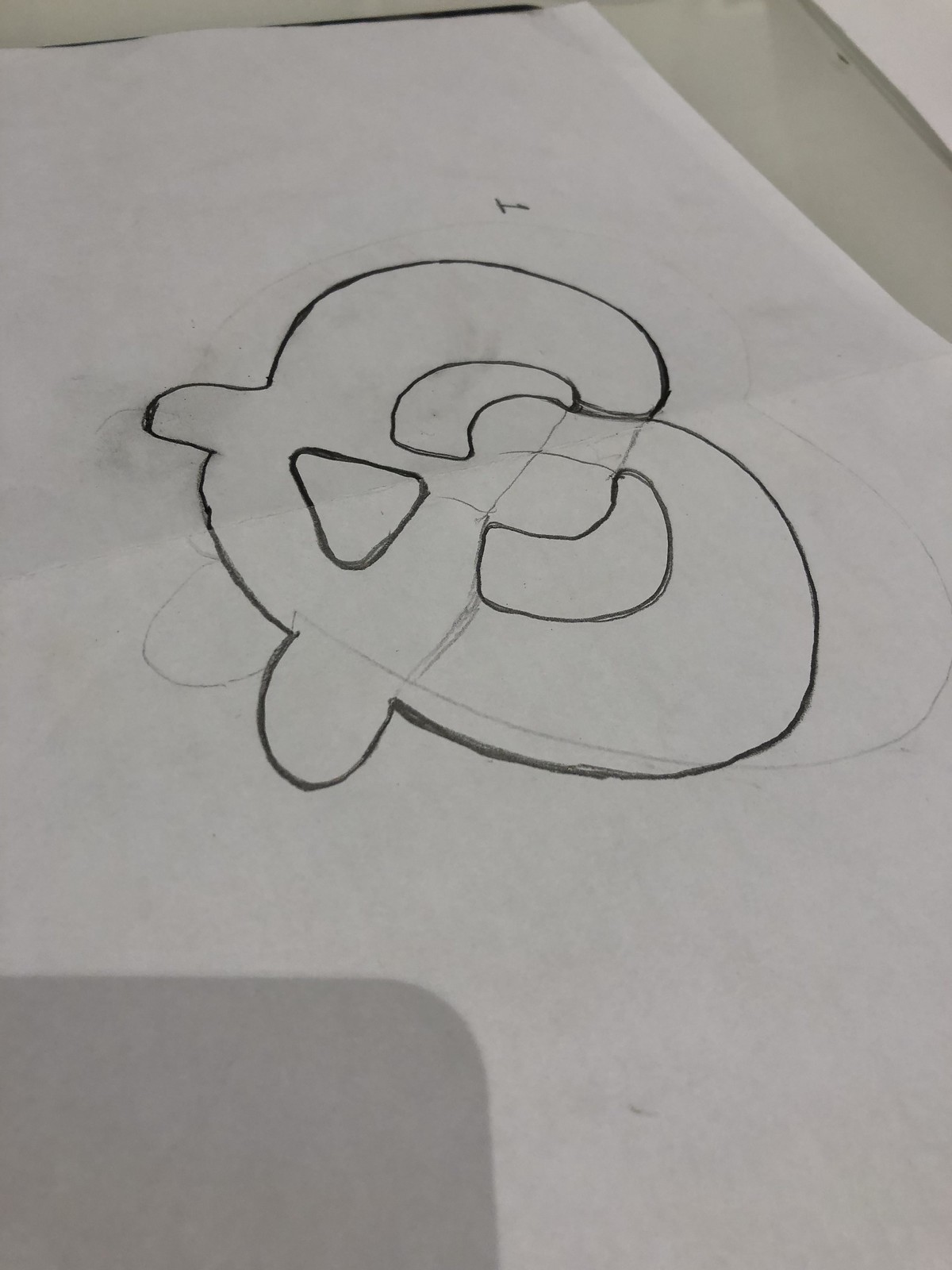The image depicts a white surface, possibly a sheet of paper or a white worktable, in the center of which there is a drawing. This drawing is quite unusual, resembling a pound sign that transforms into an abstract form with curves, protrusions, and several cut-outs. The drawing is heavily outlined, indicating it was chosen from among several preliminary sketches faintly visible on the surface. These preliminary lines suggest the artist experimented with various ideas before settling on the final design. In the lower left corner of the image, there is a square grey mat with a rounded edge, contrasting against the white surface. The edge of the white surface itself is bordered by a small strip of a creamy-colored background, potentially a wall, visible in the upper right corner. This composition creates a striking interplay between the abstract drawing and the clean, minimalistic backdrop.